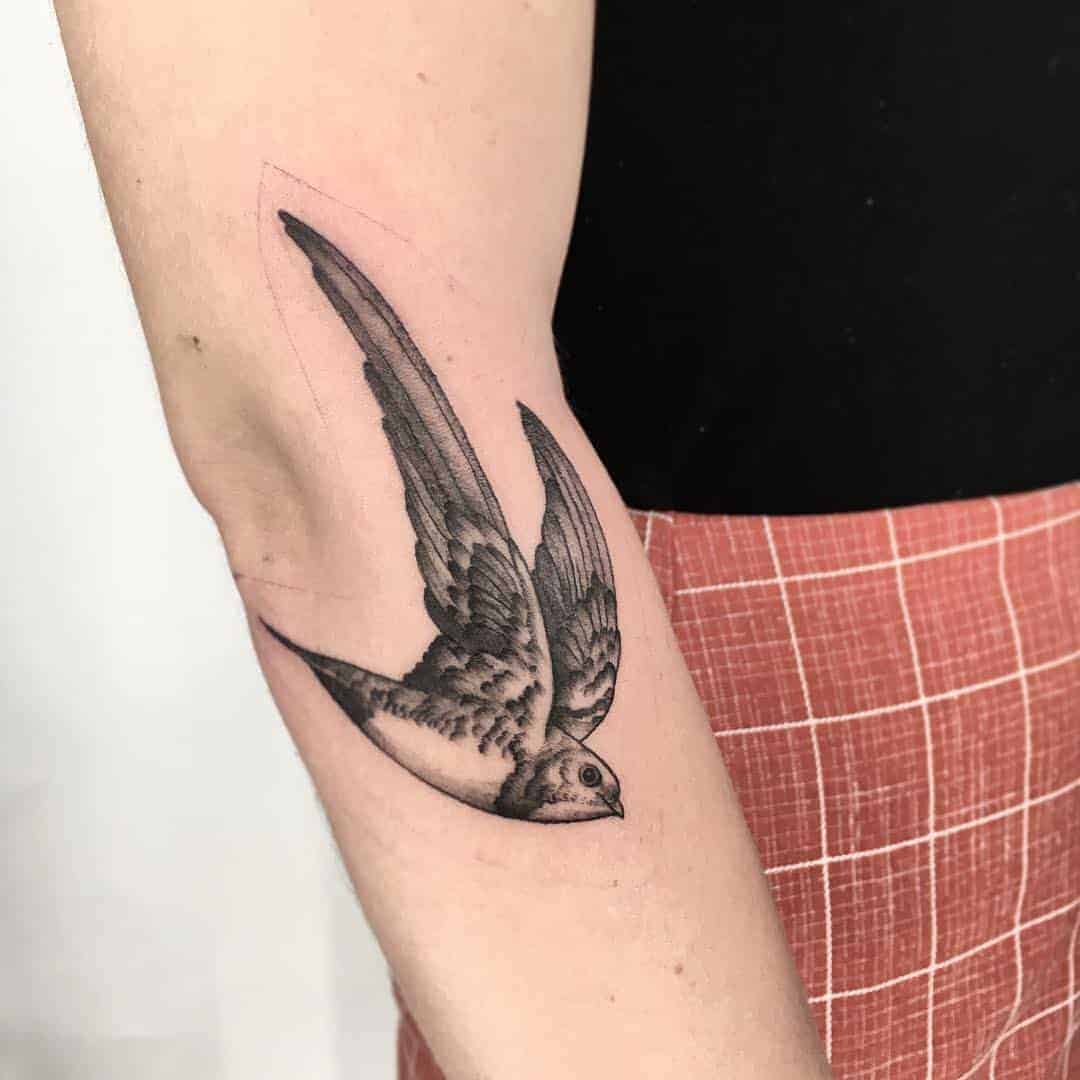The image showcases a detailed black and white tattoo on the forearm of a light-skinned person. The tattoo features a bird diving downwards with both wings arched upwards and facing towards the person's hand. The bird's intricate design includes distinct features such as an eye, a beak, a white belly, white-tipped wings, and a pointed tail. The person is dressed in a black top with bottoms that are a reddish peach color adorned with white stripes and a crosshatch pattern, which could be mistaken for a checkered brown and tan skirt. The backdrop of the image is a plain white wall, and the photograph is clear and well-lit, highlighting the details of the tattoo and the person's attire.